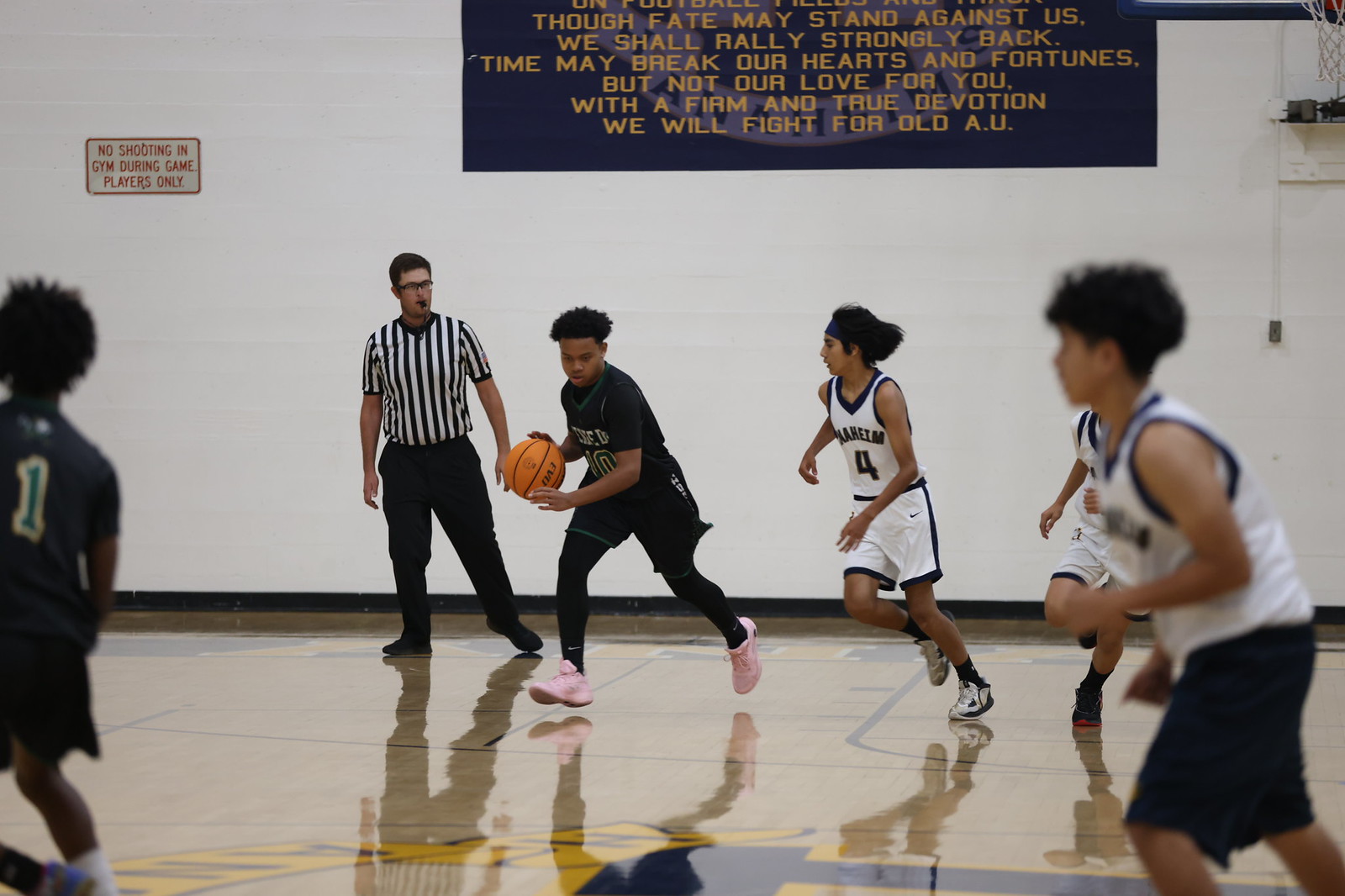In this detailed image of a youth basketball game, likely featuring players around 12 to 13 years old, the action unfolds in an inviting gymnasium with white walls and a shiny floor reflecting the players' movements. The gym is adorned with a large black banner displaying an inspiring message: "Though fate may stand above us, we shall rally strongly back. Time may break our hearts and fortunes, but our love for you with a firm and true devotion, we will fight for old AU." Another sign on the left wall cautions against unauthorized shooting during the game, specifying "players only."

The photo captures five players and a referee. The referee, distinguishable in his traditional striped shirt and dark pants, also wears glasses. The two teams are easily differentiated: one team dons black uniforms with blue stripes, while the other team wears all white. Among the black-uniformed players, one stands out in black leggings and pink shoes, adding a splash of color to the scene. The white team players have different footwear choices, including white shoes with a blue strike and black shoes with a red sole.

In the midst of the game, a player from the black-uniformed team is in the backcourt, maneuvering the basketball up the court as his teammates position themselves strategically. Three members of the opposing white team observe closely, ready to defend. The spontaneous and informal nature of the match is underscored by the slightly non-standardized uniforms. The dynamic moment has been captured in a widescreen format, emphasizing the energetic spirit and the youthful enthusiasm of the players.